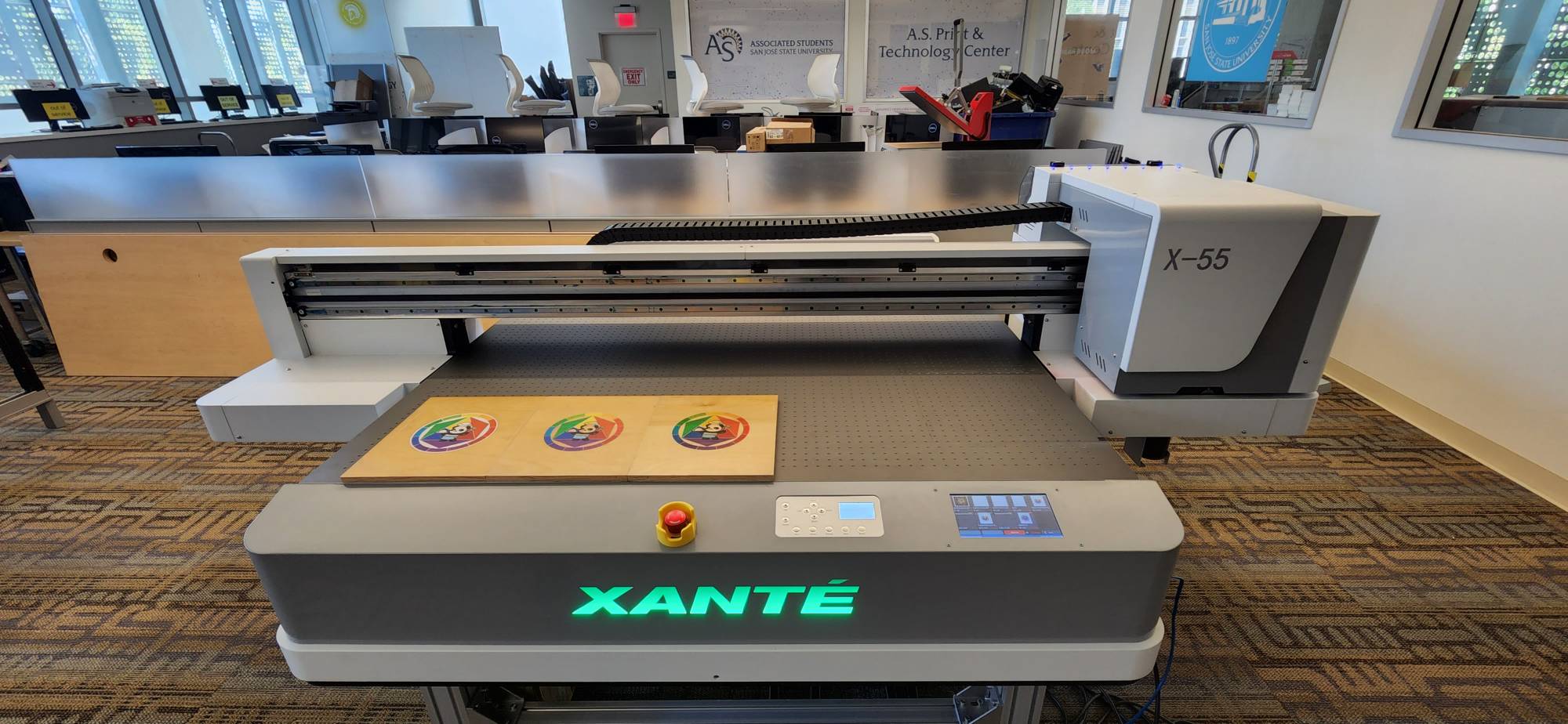The photograph captures the interior of a well-lit print and technology center, specifically within a building associated with the Associated Students of San Jose State University. Prominently featured in the foreground is a Xerox machine, labeled “X55” on the right side and marked with the brand name “Xante” in illuminated green letters spelling X-A-N-T-E. Resting atop the machine is a wooden board adorned with colorful rainbow circles in the center. Behind the Xerox machine, several computer monitors are arrayed in a row on a desk, emphasizing the organized setup of the workspace. Through the open blinds, daylight illuminates the room, complementing the indoor lighting. Part of a chair is visible on the left side, and the floor is carpeted in a mix of red and light hues, contributing to the overall clarity and brightness of the setting. Notably, the room is devoid of people, highlighting the machinery and technology on display.